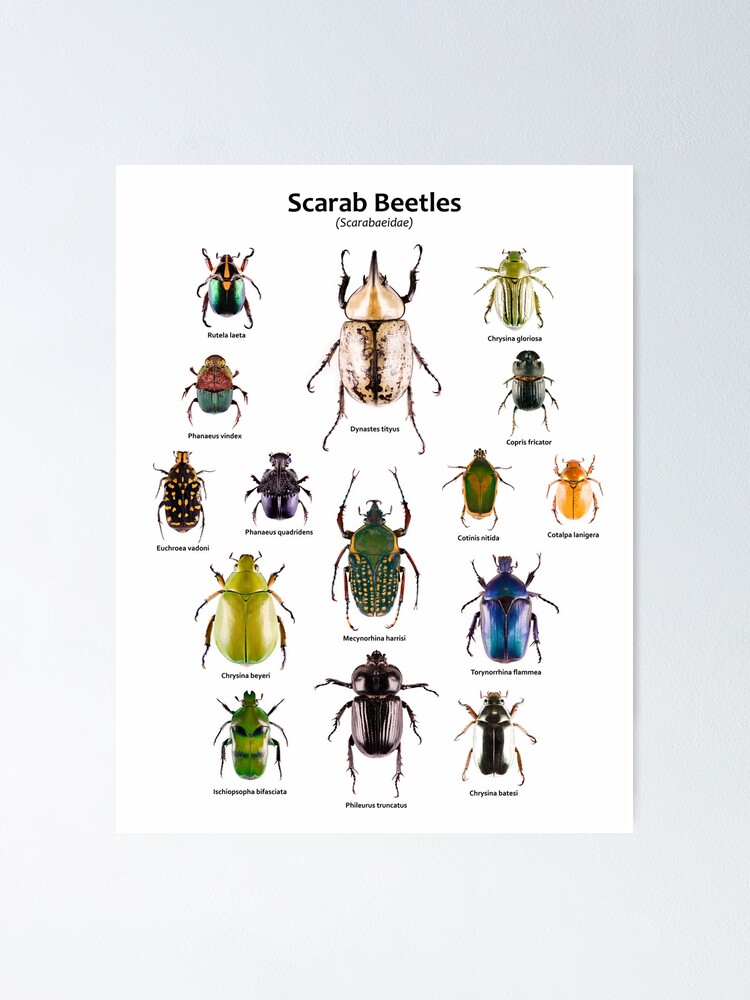The image is a detailed educational poster of scarab beetles, featuring 15 distinct beetles showcased against a light gray background. At the top, the poster is labeled "Scarab Beetles" with "Scarabaeidae" in parentheses below, indicating the Latin name. Each beetle is meticulously illustrated in vivid colors, ranging from a silver-gold beetle at the top to various shades of green, blue, black, yellow, orange, and even iridescent hues.

From the top-down and left to right, the sequence begins with the largest silver-gold beetle. Moving downward, a variety of beetles follow: a black beetle with blue and yellow markings, a striking yellow-green beetle, a smaller black beetle with spots, a gray beetle, a significant green beetle, and a diminutive green beetle. In the middle of the arrangement are two beetles colored green and black, adjacent to a shiny gray beetle and a smaller black beetle.

Further down, two distinct beetles are positioned: one green with a yellow-heart shape on its back and another yellow-orange beetle. Below these, there's a larger metallic blue beetle followed by a gray beetle with white sides. Each beetle is labeled with its respective name, though the text is not legible due to the size and clarity.

This detailed composition makes the poster a perfect educational tool, ideal for display in libraries or school classrooms, offering a comprehensive visual introduction to the diversity within the Scarabaeidae genus.